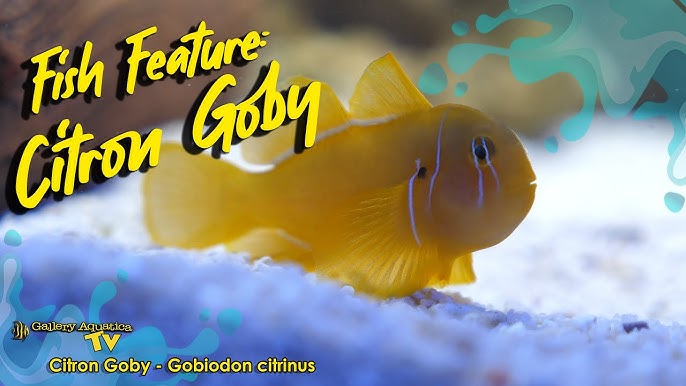The photo captures a detailed scene from an aquarium, featuring a vibrant yellow Citron Goby (Gobiodon citrinus) with striking white lines across its face, including two lines over its eye and one across its fin. The fish, which has a teardrop shape and a small black spot on its fin, is centrally positioned against a backdrop of fine white gravel, indicative of an aquarium setting. Decorative text in the top left corner, styled in yellow marker-like letters, reads "Fish Feature: Citron Goby." In the bottom left corner, there is a playful logo that says "Gallery Aquatica TV," followed by the fish's scientific name. A green splash design decorates the top right corner, adding a cartoony element to the otherwise realistic image.